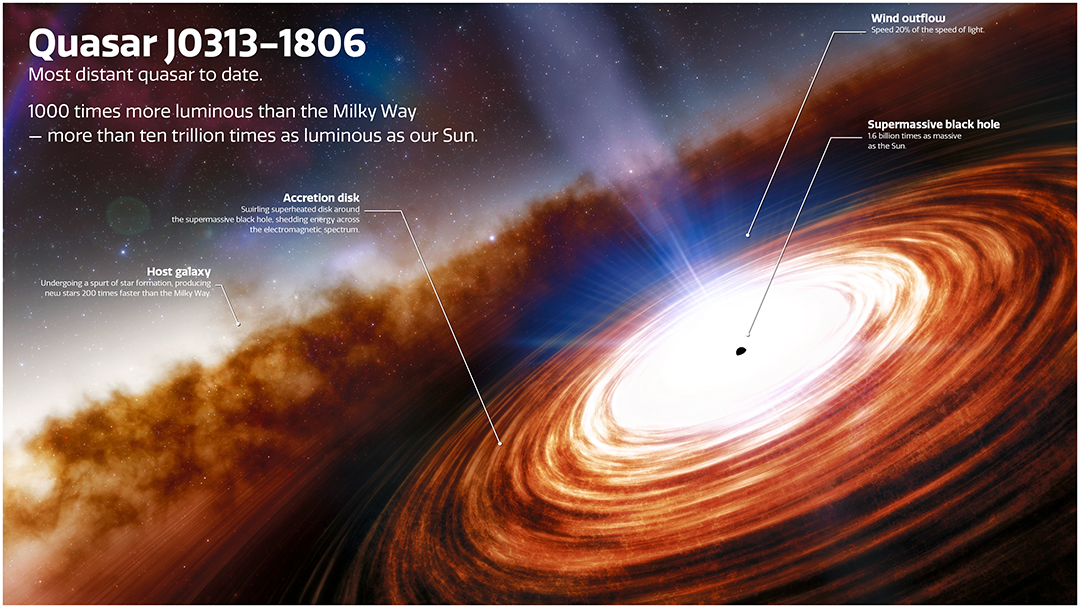This image is a detailed, computer-generated illustration of Quasar J0313-1806, the most distant quasar known to date. The quasar is depicted in the lower right quadrant of the image, showcasing a bright central spiral that transitions from white to orange, red, brown, and nearly black as it extends outward. This represents the different parts of the quasar, with the center, labeled as a "supermassive black hole," indicated by a small black dot. Surrounding the black hole, labeled arrows detail other components: "wind outflow," "accretion disk," and "host galaxy."

The accretion disk is the bright, white area near the center, which gradually turns orange and darker as it spirals outward. The "wind outflow" refers to the almost ghostly jet seen emanating from the center. The far background and upper left quadrant illustrate a starscape, giving context to the quasar's position in the universe, with numerous stars scattered across a dark expanse.

Text annotations at the top left-hand corner of the image provide key information: "Quasar J0313-1806, most distant quasar to date, a thousand times more luminous than the Milky Way, more than 10 trillion times as luminous as our sun." Although there are several small explanations under each label, they are too small to be legible. This comprehensive image highlights the quasar's astounding luminosity and structure, as well as its context within the universe.